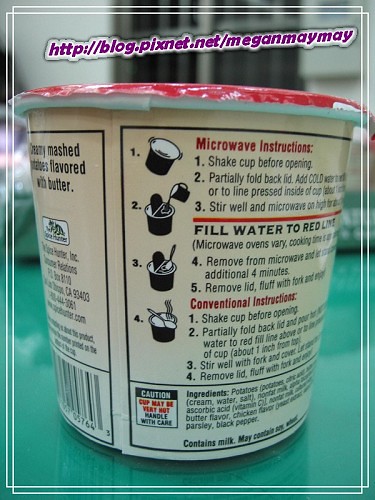The image showcases the back of a single-serving microwavable container, specifically a plastic cup retail dispenser with a plastic seal on top. This product is a microwave treat, specifically creamy mashed potatoes flavored with butter. 

Detailed instructions for preparation are provided, stating: 
1. Shake the cup.
2. Partially fold back the lid.
3. Add cold water up to the indicated line.
4. Microwave the cup.
5. Remove from the microwave and let it set for four minutes.

Additionally, conventional instructions for other heating methods are noted. The top left corner of the packaging highlights that the mashed potatoes are flavored with butter, though the word "creamy" is slightly out of focus. 

The ingredients list confirms that the primary ingredient is potatoes, accompanied by other components such as milk. There are also allergy warnings indicating the product may contain soy and wheat. A barcode is visible on the left side of the packaging.